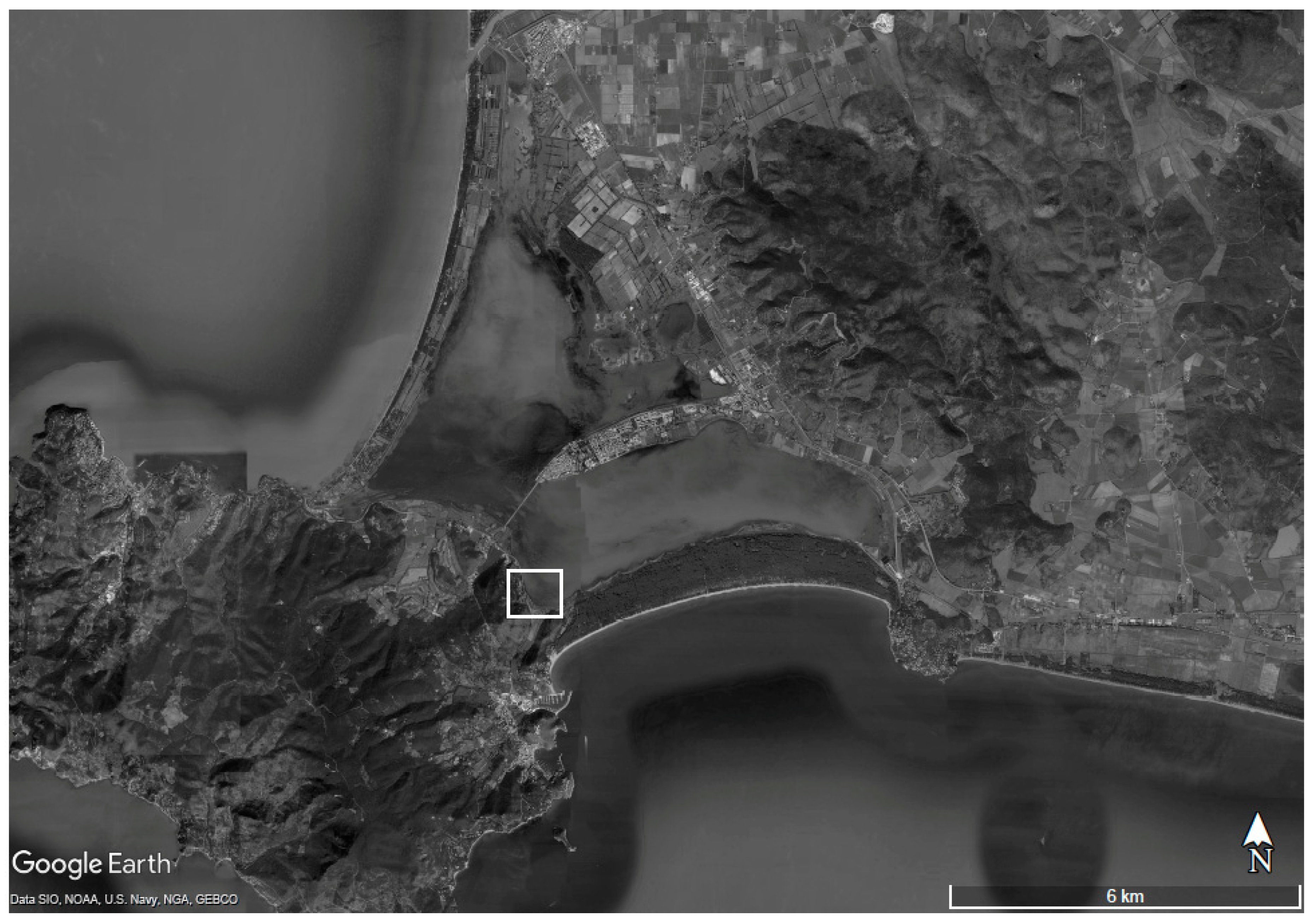This detailed Google Earth topographical image provides a bird's-eye view of rugged terrain characterized by dark, ridged areas indicative of mountains or significant elevation changes. In the bottom left corner, the image is tagged with "Google Earth, data SIO, NOAA, US Navy, NGA, GE, BCO," and features a white bracket labeled "6KM" indicating the scale, with a north-pointing arrow marked "N." The black and white image reveals a mostly uninhabitable, mountainous landscape, with what appears to be a large crater or several prominent highlands dominating the scene. Additionally, there is a small white rectangular box, not filled in, located in the bottom left quadrant, amidst the dark, ridged terrain. Near the upper middle section of the image, faint indications of structures suggest the presence of small houses or buildings, hinting at minimal habitation. Overall, the terrain appears difficult to access and sparsely populated.